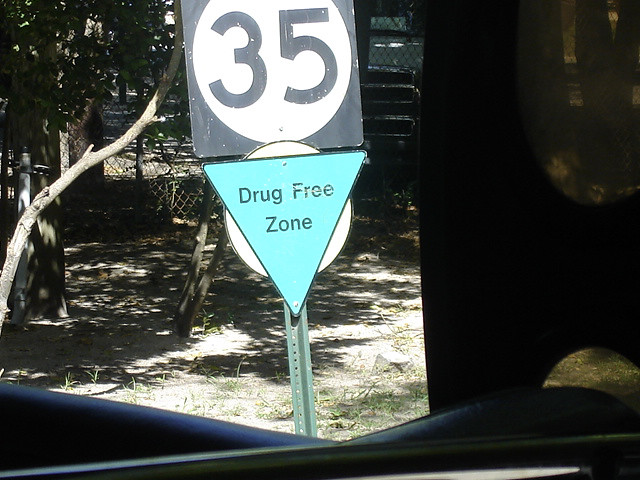The image, apparently taken from the perspective of a car window, features a roadside view with thick black framing indicative of the window's border. Dominating the center of the scene are two distinct traffic signs affixed to a thin, dark green metal pole dotted with small holes. The upper sign is a white circle with a bold black "35" at its center, surrounded by a black square. Beneath this, an upside-down triangular sign, in a bright blue hue, reads "Drug-Free Zone" in black text, set against a white circular background. Behind and around these signs, a wooded area is visible, with various trees and dense foliage creating a natural backdrop. In the distance, a chain-link fence can be discerned. The foreground features grass interspersed with patches of dirt or sand, contributing to the scenic, outdoor setting. Towards the right, indistinct shapes in shades of brown or black can be observed, partially obscured by light from the sun.